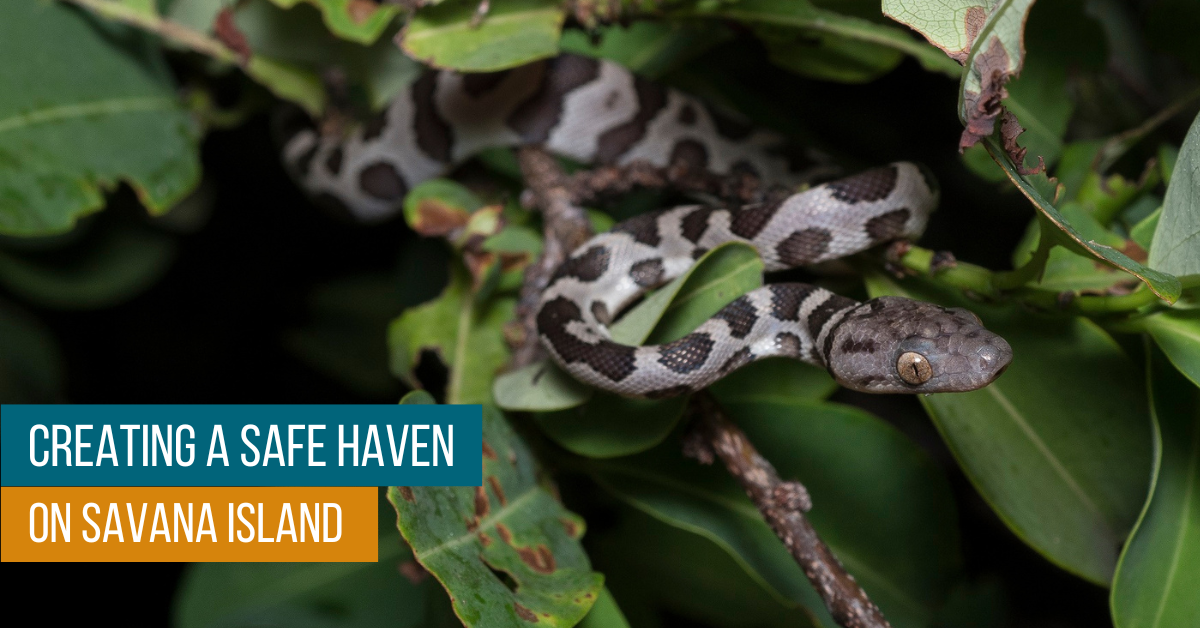This detailed image captures a close-up of a silver snake with black spots, intertwined and curved around a branch amidst glossy green leaves sprinkled with some brown, dying ones. Its body, predominantly silver with white areas between its numerous black spots, extends into a head that is a darker gray, almost concrete-like, featuring brown eyes with black pupils and smaller black spots. The snake's tail is indistinct, blending into the blurred background. In the lower left corner, two rectangles with white text stand out against colorful backgrounds: the upper blue rectangle, slightly darker, reads "Creating a safe haven," and the lower orange rectangle states "On Savannah Island." Bright daylight illuminates the scene, emphasizing the natural habitat and the snake's intricate patterns and textures.